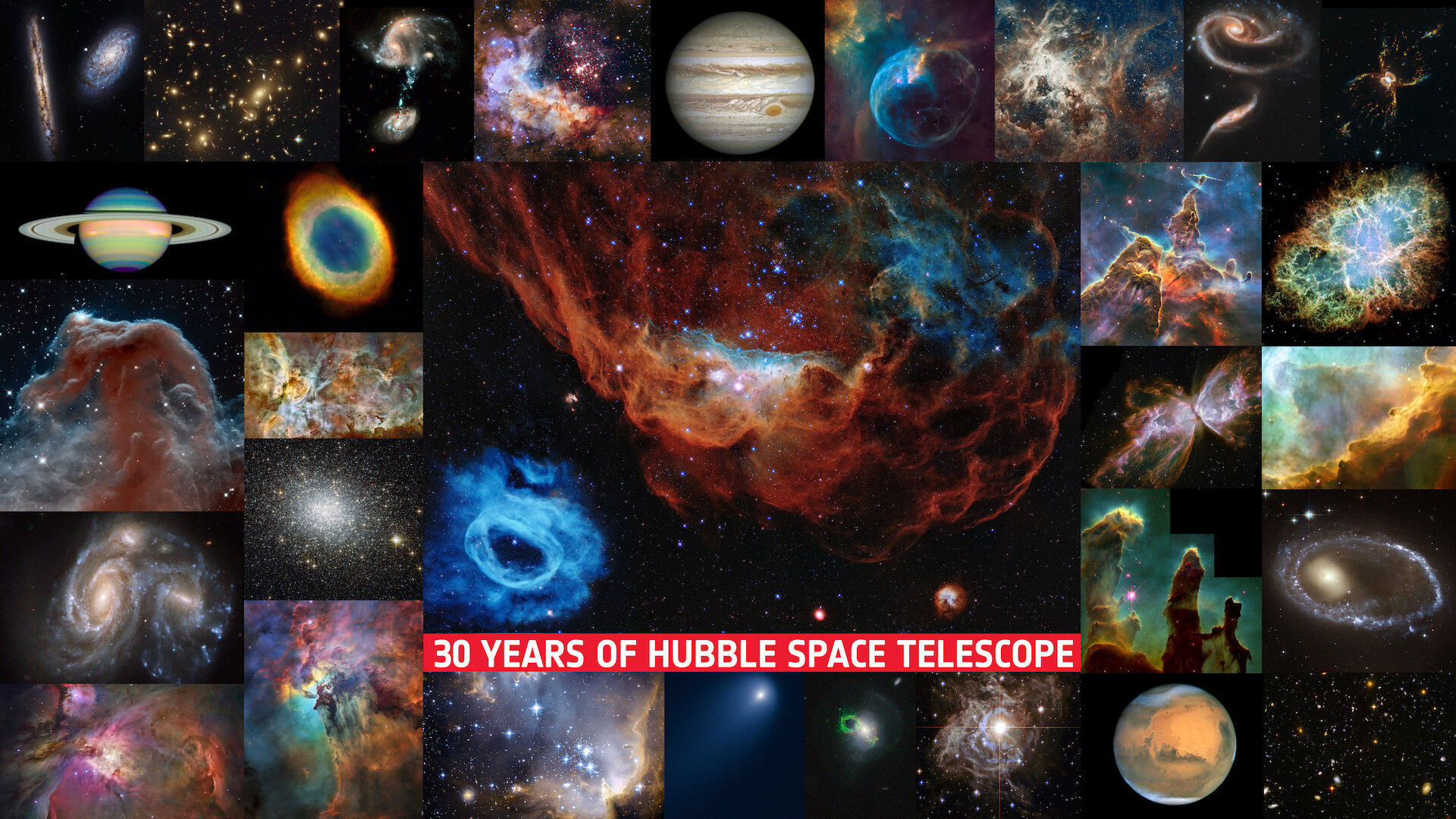The image is a vibrant and colorful collage celebrating "30 years of Hubble Space Telescope," as noted in bold white text outlined by a red box at the bottom center. The collage features over a dozen smaller pictures highlighting various celestial bodies and phenomena captured by the Hubble Space Telescope. Prominent images include a ghastly orange nebula filled with shiny stars at the center, contrasted by a smaller bluish nebula. Surrounding these are stunning shots of galaxies, stars, and planets such as Jupiter, Saturn, and Mars. The rich assortment of colors—ranging from greens and blues to tans and rainbows—showcases the diverse beauty of outer space, making for an incredibly vibrant and captivating display.